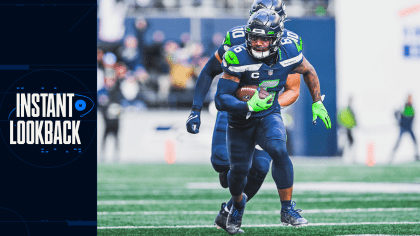A vividly detailed action shot captures two Seattle Seahawks football players in the midst of a game on a green field. The primary colors in the image are the team’s signature blue and lime green, with subtle hints of white and orange. The player in the foreground, wearing jersey number 66, is seen holding the football securely in his right arm, complemented by one blue glove and one green glove. His teammate, number 10, positioned just behind him, appears ready to block any oncoming opposition. In the blurred background, there are spectators and staff members on the sidelines, adding to the lively atmosphere of the stadium. The left-hand side of the photograph features a graphic with the text "Instant Look Back" in white against a blue backdrop, indicating a highlight moment. The image is formatted to high-definition TV dimensions, being wider than it is tall.